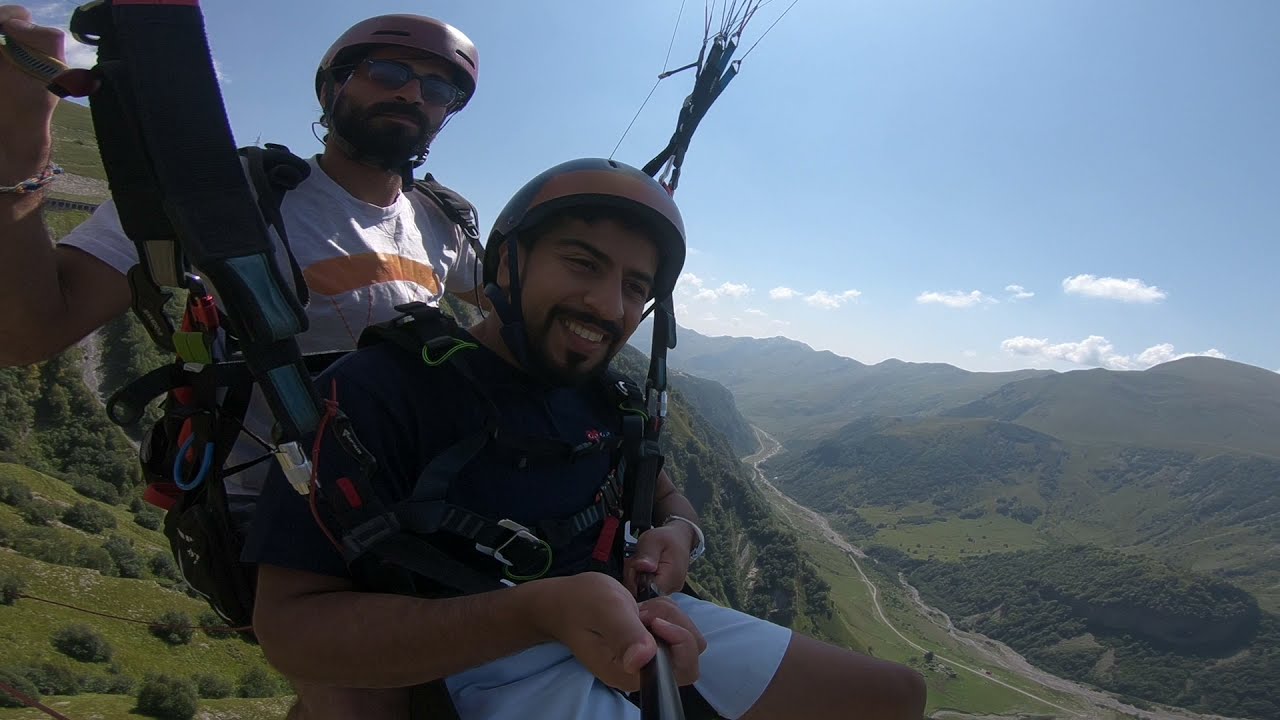In this vibrant midday photograph, two young men of likely South Asian descent are captured paragliding over a picturesque, sprawling landscape of green hills and open valleys. The man seated in front, sporting a navy blue short-sleeved shirt and light-colored shorts, holds a GoPro on a selfie stick and beams a smile as he gazes down at the grassy expanse beneath him. Behind him, the second man, wearing sunglasses and a white short-sleeved shirt with an orange stripe, appears more focused, gripping the paraglider's controls. Both wear harnesses and orange helmets, ensuring their safety as they soar through the sky. Beneath them, the rolling hills and winding roads stretch out, devoid of buildings or other people, with towering, grassy hills fading into the distant horizon. The top left corner of the image hints at a tall hill, possibly the spot from which they launched. The bright, sunny day is underscored by the clear blue sky dotted with soft, white clouds, capturing both the thrill of their adventure and the serene beauty of the landscape below. The palette of colors—light blue, various greens, and the earthy tones of the men's gear—completes the dynamic and exhilarating scene.